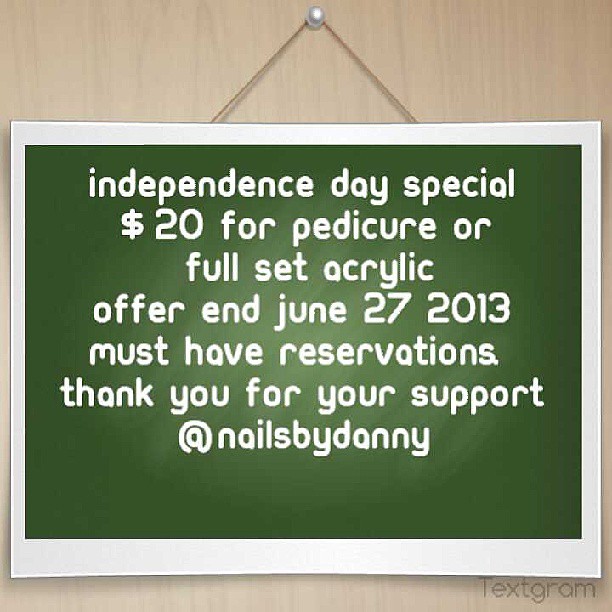This digital image, possibly downloaded from a website, presents a low-resolution, JPEG-artifacted visual which appears to be an advertisement for a nail salon named "Nails by Danny." The central focus is a rectangular green sign with a white border, giving a chalkboard-like appearance, suggesting it's framed and hanging on a wall or door, pinned with a pearl-like thumbtack. The sign features white, lowercase text reading: "independence day special, $20 for pedicure or full set acrylic offer. end June 27, 2013. must have reservations. thank you for your support. at Nails by Danny." In the bottom right corner, partially transparent text identifies it as created with "textgram." This simple yet effective graphic was likely intended for social media platforms like Twitter or Facebook to promote the salon's holiday offer.